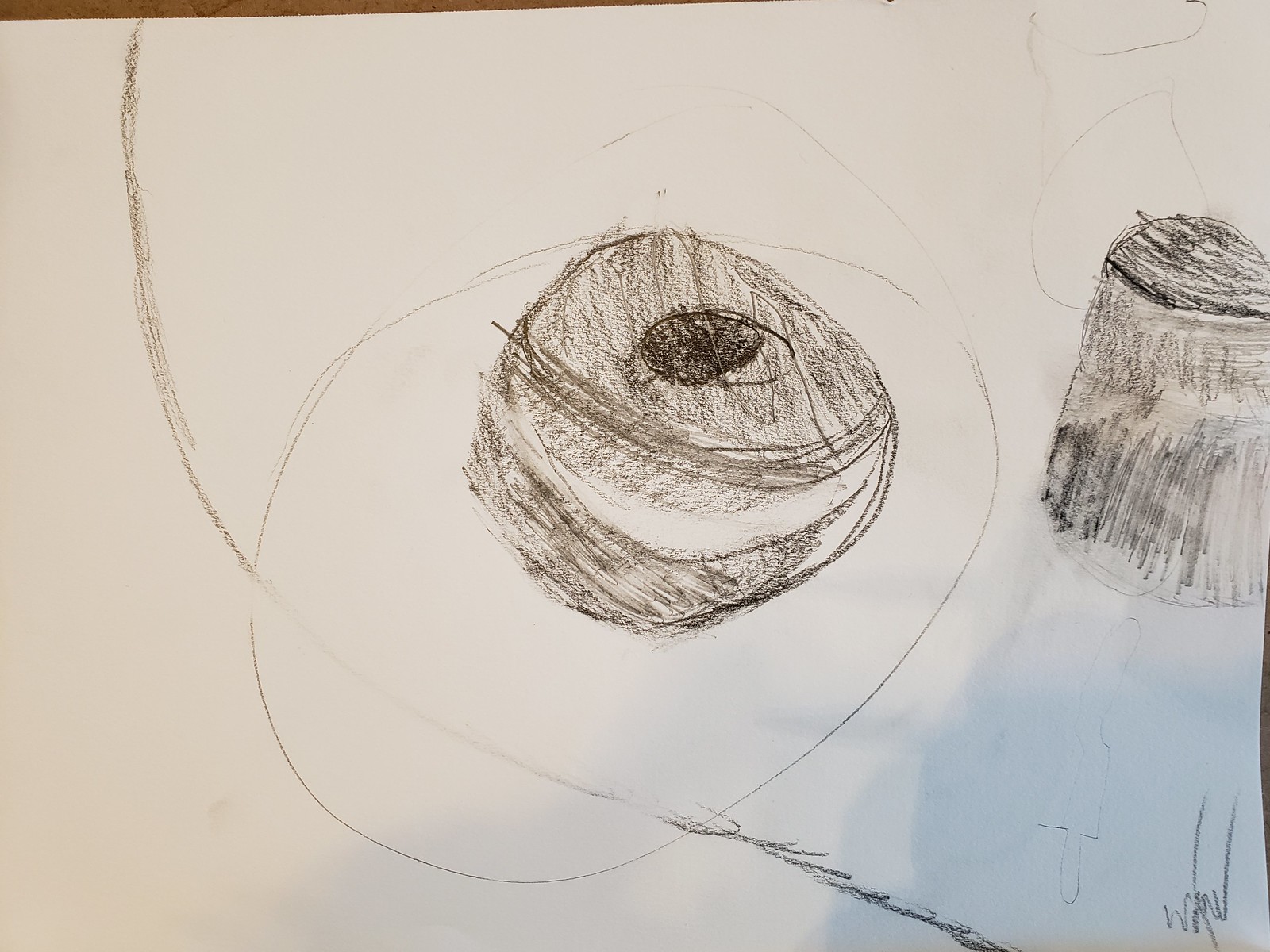This landscape-oriented photograph showcases a detailed pencil sketch, occupying the entire frame. The drawing, seemingly initialed “WMV” in the lower right corner, displays an intricate, yet indistinct scene. A central figure, circular in form, appears to be rendered with some 3D effect, potentially illustrating a small animal—perhaps a hamster—nestled within what might be interpreted as a pillow. To the right, the sketch features another ambiguous form resembling a tree stump. Surrounding these primary shapes are various other random circles and lines, contributing to the sketch’s abstract and enigmatic composition.